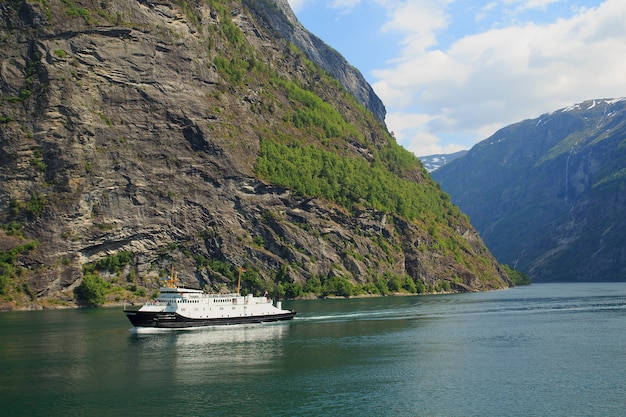This photograph captures a tranquil scene of a small cruise ship navigating through a stunning waterway, likely part of the ocean. The ship, which features a black hull and white upper structures, is situated in the bottom left-hand corner of the image. On the left side, a towering cliff face partially frames the vessel, its rocky surface adorned with patches of greenery. Further back, another rugged cliff with streaks of snow rises, contributing to the mountainous backdrop. The deep jade green-blue water reflects the crisp daytime light, under a mostly blue sky scattered with fluffy white clouds, suggesting a northern European landscape, possibly a fjord in countries like Norway or Switzerland. The overall composition showcases the ship amidst this majestic natural setting, highlighting the contrast between man-made craft and untamed wilderness.